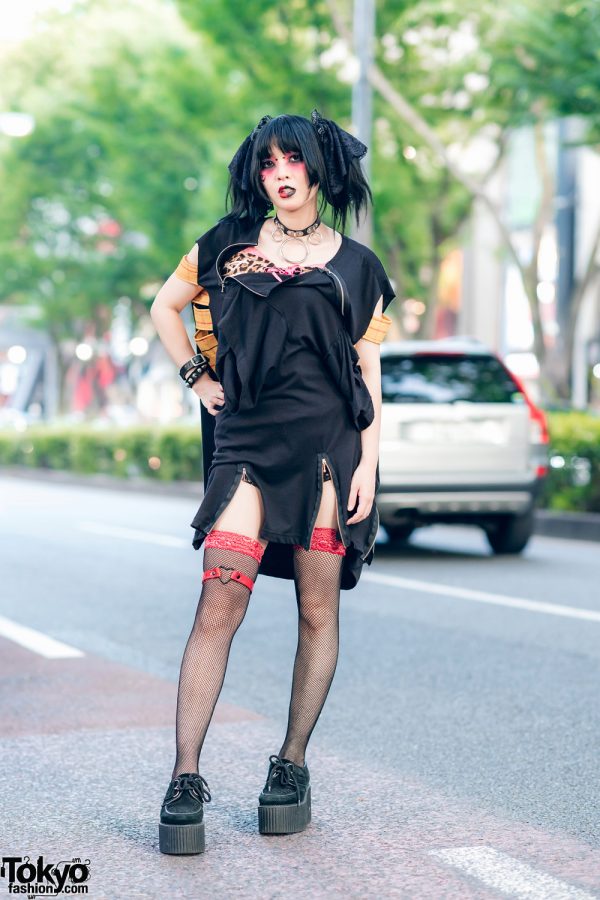In this striking promotional image for TokyoFashion.com, an Asian woman stands confidently in the middle of a blurred street, drawing all focus to her unique goth-inspired ensemble. She wears sky-high black platform shoes, black fishnet stockings topped with red garters, and an unconventional black dress that appears artfully disheveled yet non-lewd. Her accessories include a black choker and a studded bracelet, accentuating her edgy style. Her makeup is equally bold, featuring split black and red lipstick and heavy red eyeshadow. Her straight hair is styled in high pigtails, cementing her anime-inspired appearance. The text "TokyoFashion.com" is visible in the bottom left corner, suggesting this is a promotional image for the website.